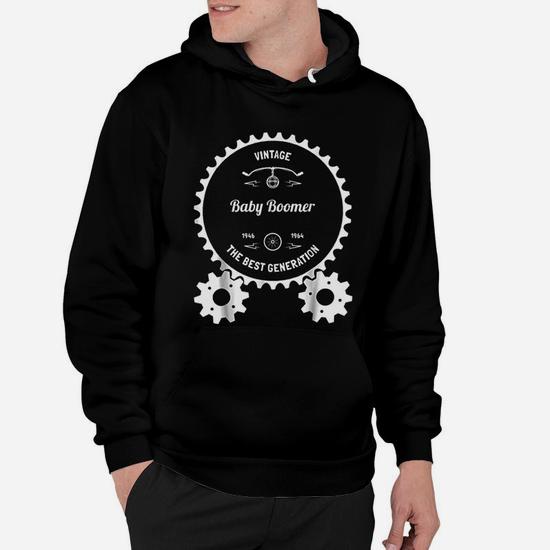The image features a close-up of a Caucasian man, who appears to be either a millennial or a member of Generation X, standing against a white background. The photo shows him from his lips down, focusing on his black hooded sweatshirt and black pants. The sweatshirt has a prominent white graphic of a large cogwheel, with the words "Vintage Baby Boomer" inside and "1946 to 1964" beneath it, along with "The Best Generation" arched along the bottom of the cogwheel. There are also two smaller gears attached at the lower corners of the larger one. His right hand is tucked into his pocket, while his left hand hangs by his side. One of the hoodie’s white drawstrings is partially visible, hanging out from the neckline.